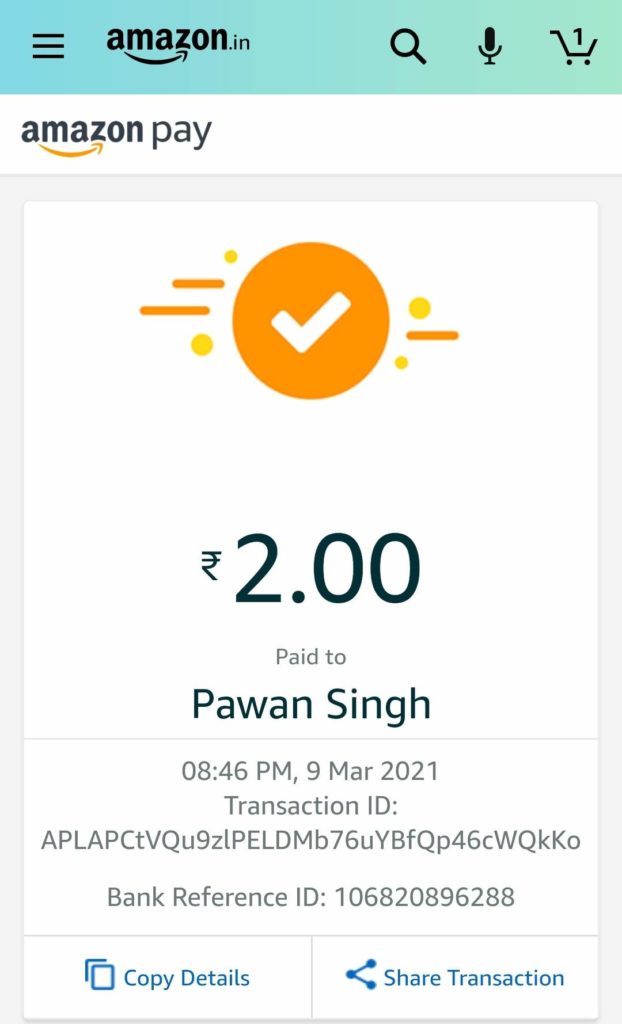**Transaction Proof for Amazon Pay**

An image displaying a screenshot of an Amazon Pay transaction summary features the following details:

- **Amazon Logo**: The top section has the familiar Amazon logo with three black horizontal lines to its left, resembling a menu button. 
- **Search Bar**: A search bar with a microphone icon and a cart icon for shopping are visible.
- **Amazon Pay Indication**: Below the logo, a prominent orange line signifies the use of Amazon Pay.
- **Transaction Status**: An orange circle with a white check mark inside it highlights that the transaction was successful.
- **Transaction Amount**: The amount paid is $2. This detail is rendered in bold, black font.
- **Transaction Specifics**: 
  - The transaction was made to "Paw on Song" at 8:46 PM on March 9, 2021.
  - A transaction ID is partially visible, starting with "applica to the q9 cc..." and "damage z7 6e...".
  - A unique reference ID: 10 168 1068 million 208 billion 962 thousand and eighty eight.
- **Copy and Share Options**: 
  - An option to copy details to blue pages is mentioned, along with a share button symbolized by a blue icon.
  - The vendor's name "Paw on Song" is displayed in black or blue writing, with the $2 amount highlighted in bold black text.

The composition of the screenshot captures the detailed administrative and financial aspects of a small digital transaction, emphasizing the security and convenience of Amazon Pay services.